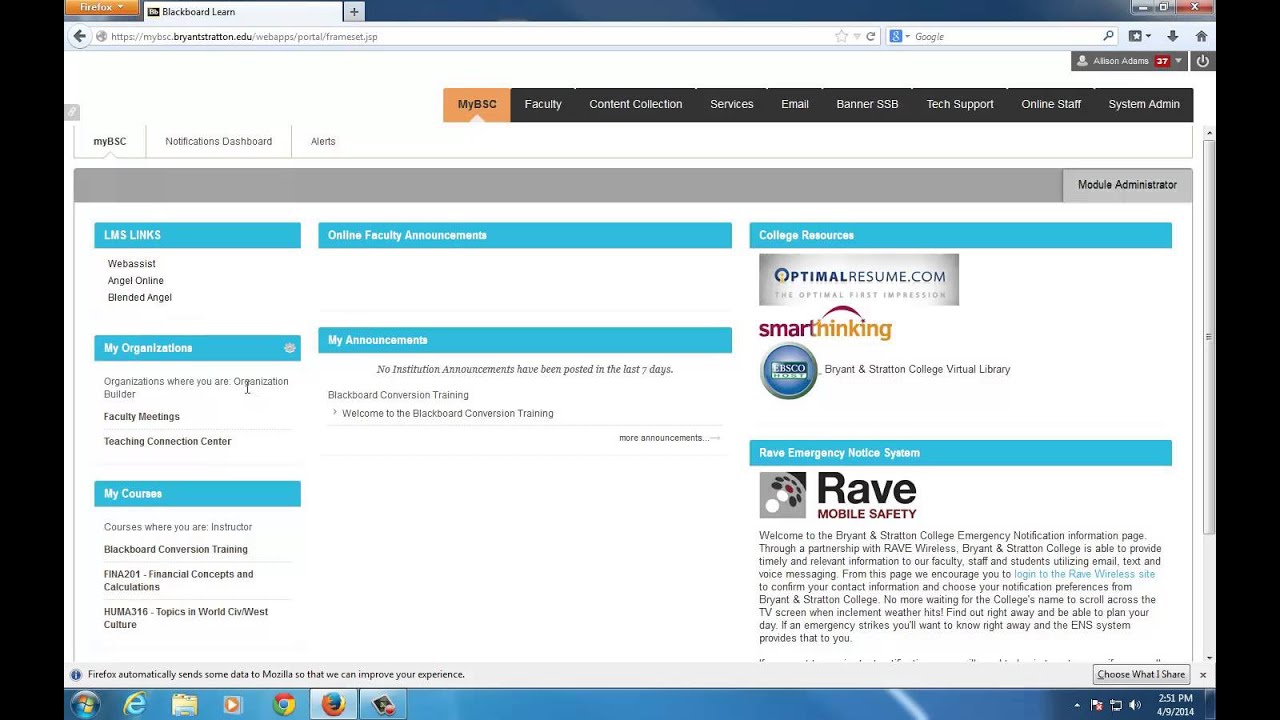The screenshot portrays a computer interface with notable features and elements captured in great detail. A black strip runs vertically down both the left and right sides of the screen. In the upper left-hand corner, an orange button is prominently displayed.

Moving to the top right, the controls for minimizing, closing, and enlarging the window are visible but partially cut off. Below this, the address bar is situated with a black arrow icon on the far left. Towards the right of the address bar, there is a search bar accompanied by several additional icons.

Approximately three lines down from the top, a menu bar is visible starting slightly left of the center. The menu items include: an orange-highlighted "ESC" or similar acronym, followed by black tabs with white text displaying options such as Faculty, Collection, Services, Email, an unreadable item, Tech Support, Online Staff, and System Admin.

Underneath this menu bar, a white rectangular section holds three tabs, with the leftmost one labeled "my" or "SEC," though it remains blurry and indistinct. Following is a horizontal gray line leading to a Module Administrator button. 

Below this, several aqua rectangles with white text stretch horizontally across the screen. The leftmost rectangle contains three listed items beneath it. Below these, two additional rectangles each with their own listings are found, with one more rectangle on the left displaying another set of items.

Adjacent to these, on the right side, various elements are displayed. There is an advertisement for "optimalresume.com," followed by logos for "Smart Thinking" and "Bryant & [unreadable] College." Further down, another aqua section appears, beneath which is a "Rave Mobile Safety" label accompanied by its icon and a paragraph of small text below it. This detailed layout captures the various interactive and informative elements of the user interface in question.